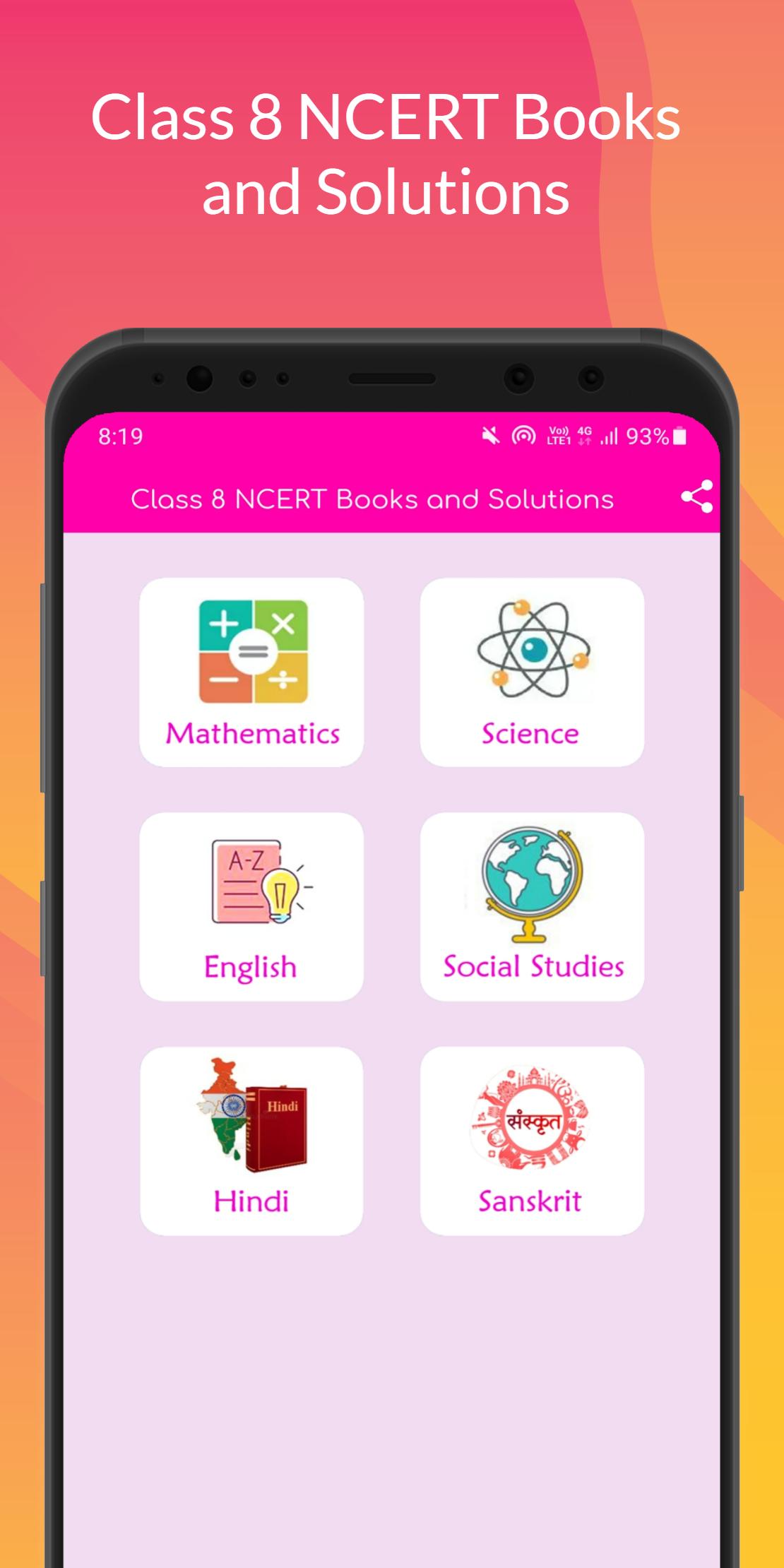The image features a gradient background starting with pink in the upper left corner, transitioning to orange in the middle, and fading to yellow towards the bottom. At the top of the image, white text boldly reads "Class 8 NCERT Books and Solutions." Below the text, a smartphone with a black case is prominently displayed. On the right side of the phone, there is a visible power button, while the left side houses the volume up and down buttons. The top of the phone's screen showcases a pink border, with the time "8:19" visible on the upper left and a battery icon on the upper right indicating a 93% charge.

The phone screen displays a lighter pink background with six white squares arranged neatly. The top left square is labeled "Mathematics" and features a calculator icon. To its right, another square labeled "Science" is marked with an atom icon. On the next row, the square on the left is labeled "English" and includes icons of a book and a light bulb. To its right, the "Social Studies" square is identified by a globe icon. The bottom row has two squares: the left one is labeled "Hindi" with icons of a brown book and a map, and the right one is labeled "Sanskrit."